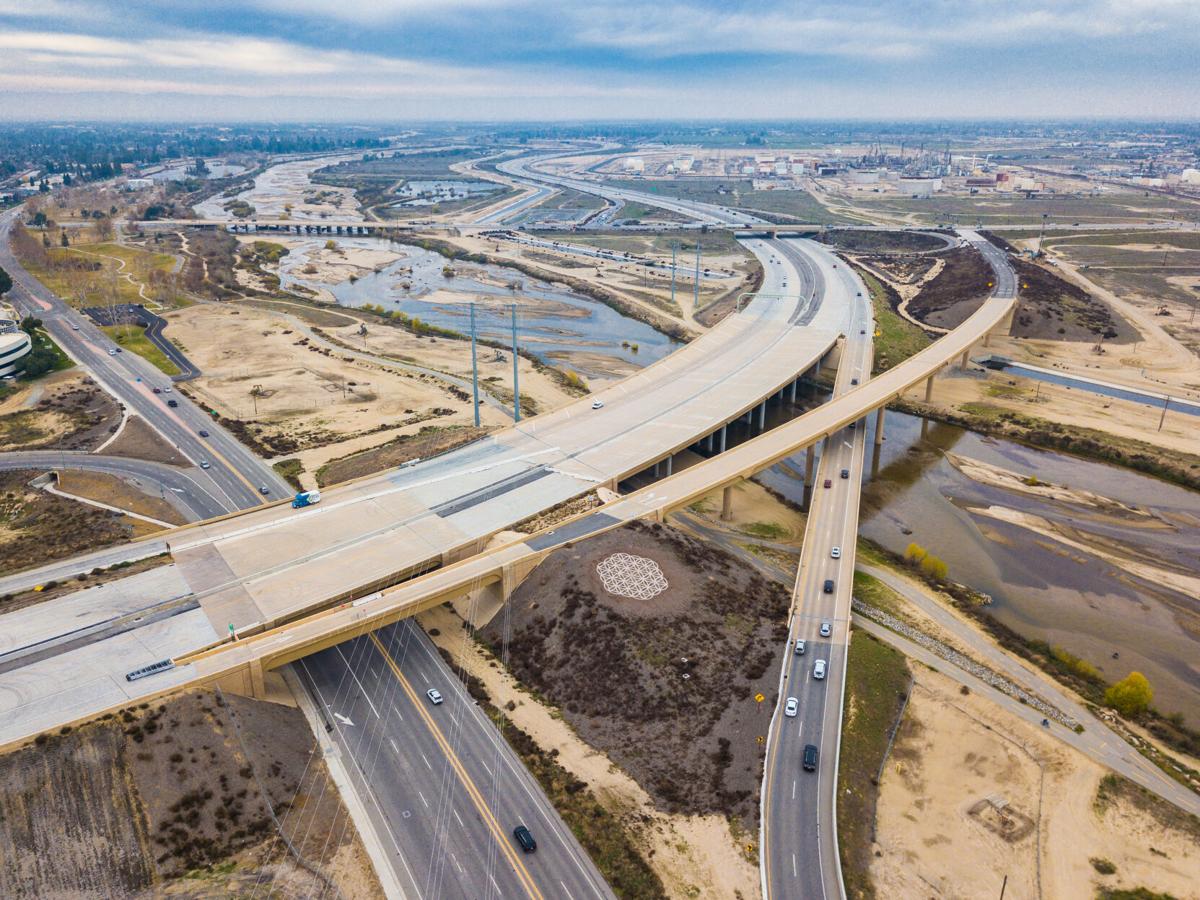This panoramic aerial view captures an extensive freeway network cutting through a dry, barren landscape. The main thoroughfare, a broad roadway with four to six lanes, runs north to south, intersecting with various other roads and elevated flyovers. In the heart of this arid terrain, there's a captivating lattice-like geometric design, possibly representing a Garden of Life pattern, set amidst the predominantly brown and beige farmlands. Toward the center-right of the image, a partially dried-up riverbed exposes dirt and sand beneath towering bridges. The sparse vehicles on these elevated roads contrast with the busier lower thoroughfares. Distantly, a hazy cityscape looms under a sky dotted with clouds, hinting at an impending rain despite the overall dryness. The background mixes shades of green, blue, and yellow, with sparse vegetation, industrial structures, and residential areas scattered throughout the expansive, somber scene.